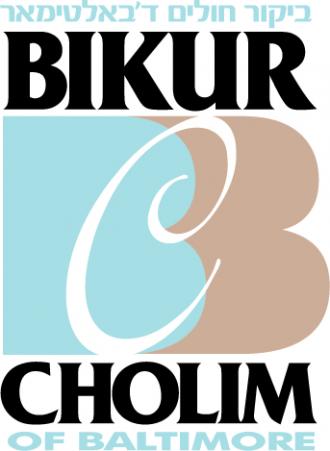This color photo showcases an intricate logo design prominently featuring a mix of text and imagery. At the top, there is a line of text in a non-English language, rendered in blue. Beneath this text, in bold black letters, is the word "BIKUR," spelled out as B-I-K-U-R. Below "BIKUR," the core logo is depicted: a stylized bee, split into two halves. The left side of the bee is a light turquoise blue, and the right side is a peachy or purple hue, with each section forming a smaller bee shape within the larger silhouette. Dominating the center of the logo is a large, white cursive “C” that intersects both colored sections of the bee. The text "CHOLIM" appears below this logo in bold black letters, followed by "of Baltimore" in blue lettering. The text "Cholim" and "of Baltimore" collectively read as "Bikur Cholim of Baltimore," tying the elements together into a cohesive representation of the organization.